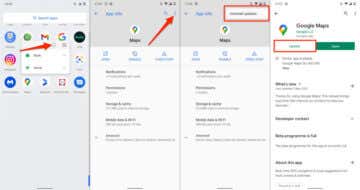In the image, there are four side-by-side screenshots of a phone screen. The screenshots are very blurry, making it challenging to discern specific details or words clearly.

**First Screenshot:**
- The background is predominantly gray.
- There is an arrow pointing to a location below the row containing the Google and Gmail icons.

**Second and Third Screenshots:**
- Both have similar, albeit blurry, backgrounds, suggesting they are almost identical.
- The third screenshot features a red box highlighting two black words, though the words themselves are unreadable due to the blurriness.
- There is a red arrow in the second screenshot pointing towards a section with two blue elements, contrasted against the red-highlighted section in the third screenshot.

**Fourth Screenshot:**
- Likely related to Google Maps, as evidenced by the visible Google Maps symbol and partial legible text that includes letters "G" and "N."
- Two colored boxes are present: one white box with green text, and another green box with white text. The exact content of these boxes is unclear, but they are highlighted with red boxes for emphasis.

Each screenshot is marked with indicative arrows and boxes, attempting to guide the viewer's attention to specific areas despite the overall blurriness and poor readability.